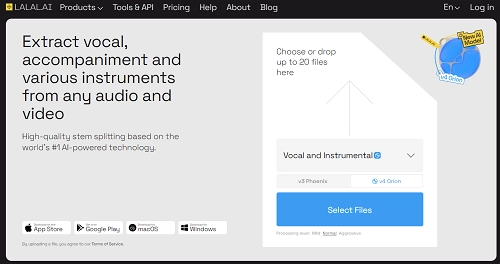The image presents a mock-up of a web page interface. It starts with a black outline surrounding the content, resembling a typical website layout. At the top, written in gray font, are the words "la, la, la, la, one." Below this, a navigation menu lists "Products," "Tools," "API," "Pricing," "Help," "About," and "Blog." To the far right of the navigation menu, options for language selection represented by "EN" with a downward arrow and a "Login" button are displayed.

The main section has a gray background with the left side text in black font. It reads, "Extract vocal accompaniment and various instruments from any audio and video," followed by a smaller font text, "High-quality stem splitting based on the world's number one AI-powered technology." Below this text are logos for the App Store, Google Play, Mac OS, and Windows.

To the right, occupying almost a square space, there's a white background box with gray font instructions: "Choose or drop up to 200 files here," accompanied by a gray upward-pointing arrow. Directly below this, on a gray background, in black font, are the options "Vocal and instruments," with a gray downward-pointing arrow next to it.

Further below, there's another gray and white box with very small font inside. A blue box contains the text "Select files," with some additional information in gray lettering beneath it. In the top right corner, there's a blue circle featuring a yellow flag to the right, a yellow banner to the left, and a white banner underneath it, divided by a gray line traversing the circle, giving it a dripping effect.